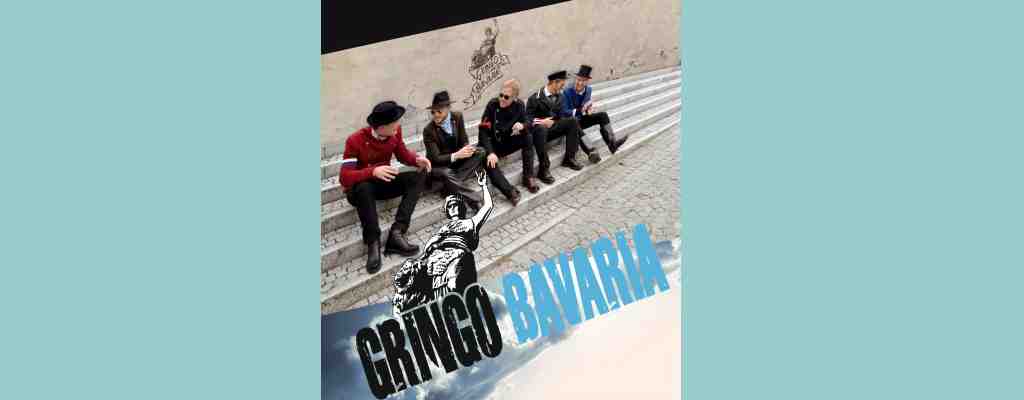The image resembles an artistic album cover set on a rectangular, teal blue poster. At the center, there is a square photo featuring five men dressed in rock star attire, complete with leather boots and hats, sitting casually on white stone steps. The backdrop displays a brick or concrete wall with graffiti, including a stylized, black and white drawing of a woman with her arm raised, reminiscent of the Statue of Liberty but more abstract and artistic. This same image of the woman appears above the text overlay at the bottom. The text "Gringo Bavaria" is slanted upward, with "Gringo" in black and "Bavaria" in blue, likely signifying a band or a logo. The scene appears to be outdoors, contributing to the rugged, rock star aesthetic.